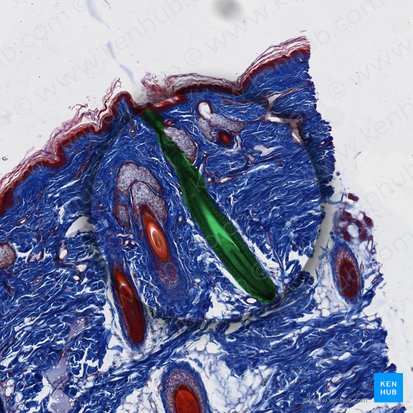The close-up photograph, taken through a microscope, showcases an intricate cell structure with a rich palette of colors and shapes. The image is rectangular, bordered by equal lengths on all sides. Dominating the bottom right corner is a blue square watermark with white text reading "Kenhub." A semi-transparent gray watermark reading "www.kenhub.com" runs diagonally from the bottom left to the top right, repeating across the image.

The vibrant composition features a predominantly angular blue background, interspersed with various white lines and red circles. A central, oblong, leaf-shaped green section contrasts with the surrounding colors. Additional orange spots and blue wavy lines add to the complexity of the visual. The periphery of the image includes a dark purple outer layer, contributing to the overall depth and layers of the photograph.

Approximately 90% of the space is occupied by these colorful details, set against a white background. The hues utilized range from royal cobalt blue, which appears almost purple, to greens, reds, whites, and grays, enhancing the dynamic and abstract nature of the subject. The red elements are more concentrated towards the edges and sporadically in the middle, while the solitary green section is prominently central.